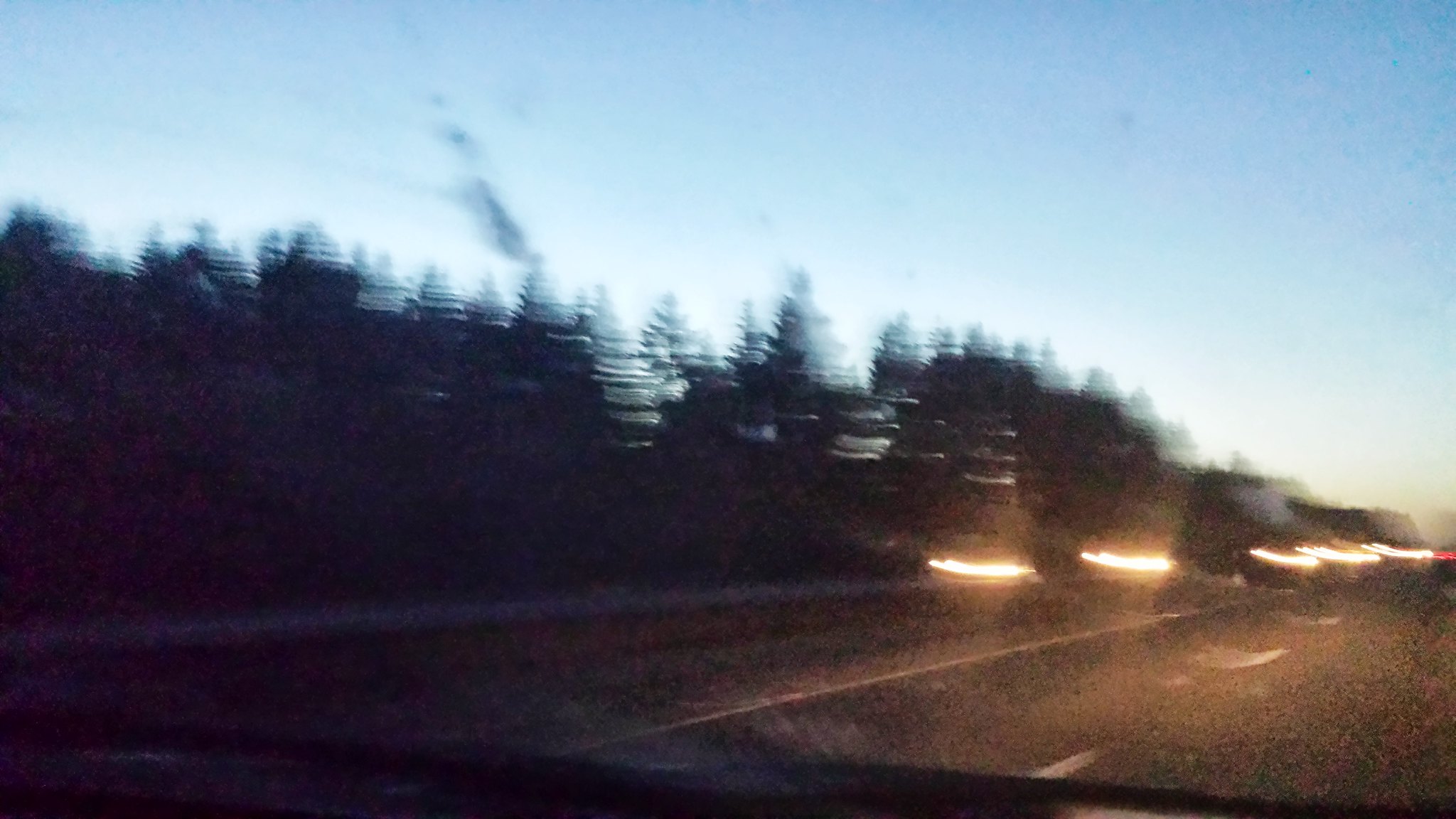This image depicts a roadway captured in a dim light setting, neither overly bright nor entirely dark. The scene is lit by an array of lights that appear somewhat ambiguous in nature; they resemble bumper-to-bumper flying saucers due to their round shape, rather than typical car headlights. The photograph seems to have been taken from within a vehicle, though the overall realism of the picture is questionable. The road itself is marked by a visible divider and unconnected white lines, presumably as lane markers. In the far distance, a red light can be seen amidst these road markings. Flanking the roadway are towering evergreen trees, suggesting a forested or rural setting. Additionally, the ground exhibits a lightness that hints at a possible dusting of snow. However, the image suffers from poor detail and blurriness, making it difficult to discern and describe features with certainty.